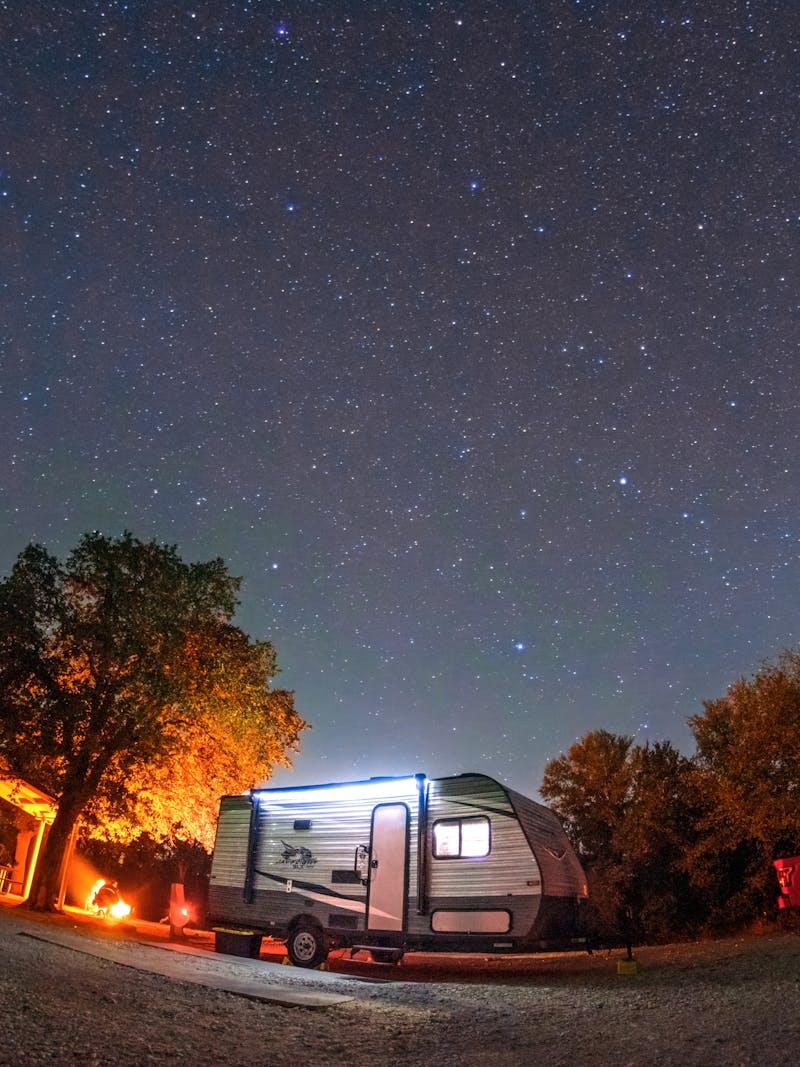The image captures a scene during a beautiful, star-speckled evening, presented in a vertically-aligned rectangular (portrait) orientation. Dominating the center of the picture is a small, tow-behind camper angled slightly with its front right corner closer to the viewer. The camper exhibits a lit interior through its two illuminated windows and is parked in what appears to be a gravel lot, adjacent to a piece of plywood or a concrete pad.

Flanking the camper on either side is a mix of trees, with a particularly large tree standing to the left rear of the camper. Below this tree and slightly behind it, a faint campfire and possibly a lean-to or canopy can be discerned, adding to the rustic ambiance. To the far right, a dense forest lies, creating a dark backdrop that emphasizes the illuminated spots and evening sky.

The sky itself is a mesmerizing display, transitioning from a lighter hue near the horizon to a darker, night-time canvas above, adorned with countless bright stars and a scattering of slightly larger, light-blue speckles. The overall landscape at the bottom of the image appears uneven and somewhat distorted, featuring a mixture of dirt and dead grass. Scattered throughout the scene are small, yellow spotlights emerging from the ground, subtly illuminating portions of the terrain and adding to the enchanting, serene atmosphere of this picturesque evening.